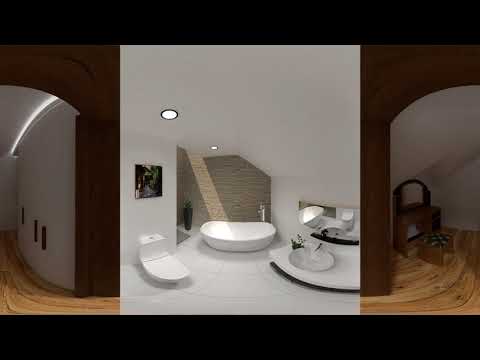The image is a color photograph displayed in portrait orientation, inset against a landscape backdrop of itself with black borders on the top and bottom. The central image showcases a modern bathroom with predominantly white decor. Dominating the center is a kidney-shaped white bathtub set against a backdrop of brown, bamboo-textured tiles. To the left, an elongated, decadent white toilet stands under a square painting. Adjacent to the tub's right is a clear circular basin atop a white countertop and dark wood cabinet, accompanied by a small mirror mounted on the wall. Overhead, recessed lighting brightens the space. Framing the bathroom, white walls extend into adjacent hallways with black or brown wooden floors, and brown wooden archways are visible on either side. The photograph captures a high level of detail with slight curvature, characteristic of photographic representationalism realism.